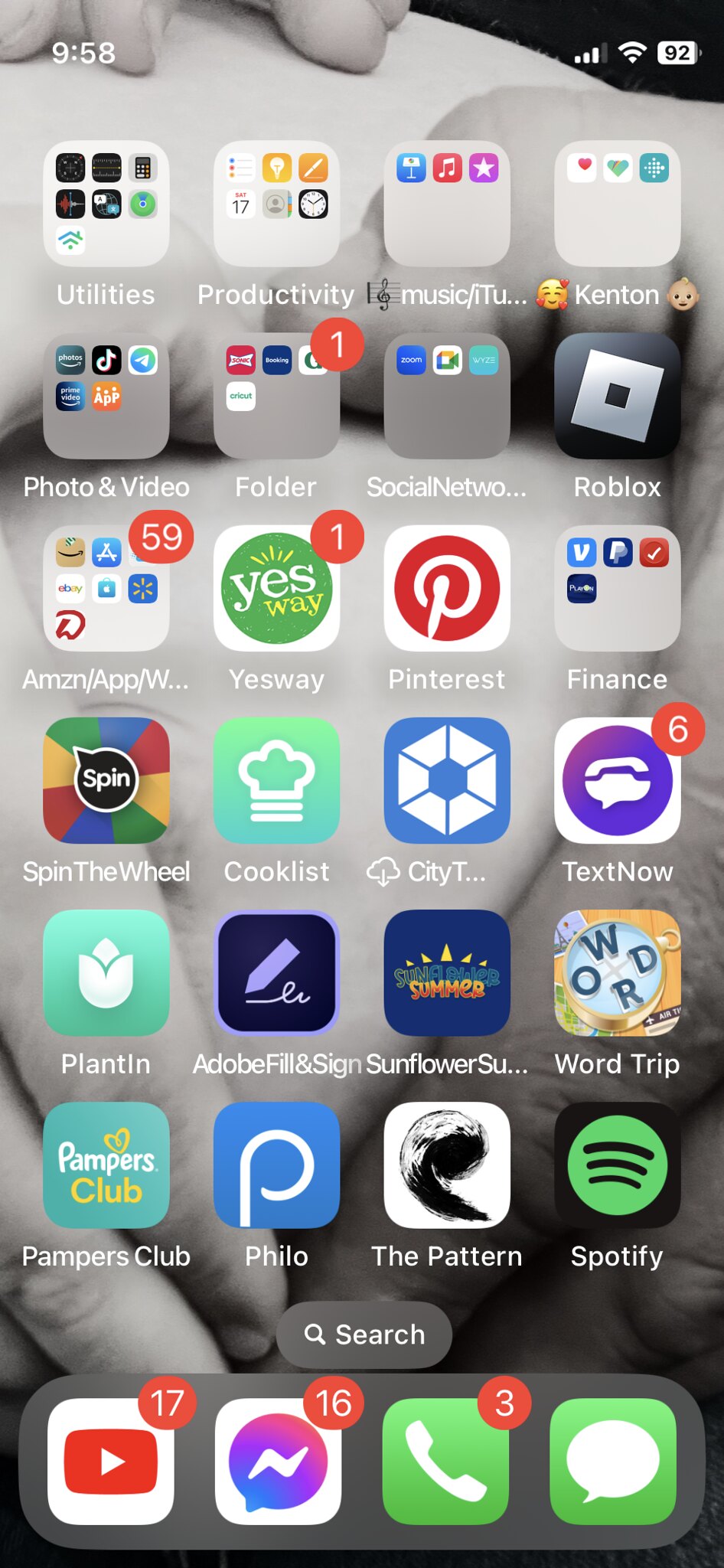A screenshot of a smartphone's homepage reveals a black and white wallpaper depicting two hands intertwined, visible at both the top and bottom of the screen. The timestamp at the top of the image reads 9:58, accompanied by an indicator showing three bars of signal strength, a data connection symbol, and a battery life at 92%. 

The first row of app folders includes:
1. **Utilities** - filled with numerous apps.
2. **Productivity** - also containing multiple apps.
3. **Music/Tunes** - holding three apps.
4. **Kenton** - featuring three apps, labeled with icons of a heart and a baby.

The second row features:
1. **Photos and Videos** - folder with several apps.
2. **Folder** - contains various apps and one notification marked by a red circle with a white "1".
3. **Social Networks** - folder with apps.
4. **Roblox** - standalone app.

The third row displays:
1. **Amazon** - shows 59 notifications.
2. **Amazon App/W...** - folder with several apps.
3. **Yes Way** - standalone app with one notification.

The fourth row includes:
1. **Pinterest** - a standalone app.
2. **Finance** - folder likely containing apps such as Venmo and PayPal.

On the fifth row:
1. **Spin the Wheel** - a game.
2. **Cook List** - an application.
3. **City...** - an app with partial name visible.
4. **TextNow** - application with six notifications.

In the sixth row:
1. **Platinum** - an app.
2. **Adobe File and Sign** - an app.
3. **Sunflower...** - likely a game with a partially visible name.
4. **Wordcher** - an app, potentially a game.

On the seventh row:
1. **Pampers Club** - an app.
2. **Filio** - an app.
3. **Pattern** - an app.
4. **Spotify** - a music streaming app.

At the bottom of the screen are:
1. **YouTube** - with 17 notifications.
2. **Messenger** - with 16 notifications.
3. **Phone Calls** - indicated by three notifications.
4. **Messages** - the default text messaging app.

Overall, this detailed view showcases a well-organized yet heavily notified smartphone screen, reflecting a busy digital life.